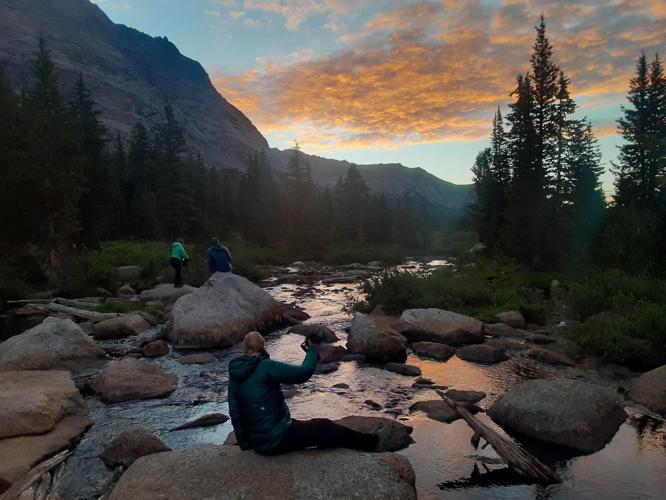This stunning color photograph depicts a serene mountain creek scene at dusk. The sky is a beautiful gradient of light blue with clouds accented by orange shadows, suggesting a setting sun. To the left, dark green pine trees stand tall against the backdrop of majestic mountains with a sandstone hue. On the right, additional pine trees frame the scene.

In the center of the image, a large river flows, filled with gigantic rocks that dwarf a person. Two figures stand on one of these rocks in the background; one wears a light green jacket and dark pants, while the other dons a dark-colored shirt. Both appear absorbed in their natural surroundings, facing away from the camera.

Closer to the foreground and towards the bottom middle of the image, another person is waving their right hand. This individual is clad in a dark green puffer jacket, complemented by pants and tennis shoes. The entire group has their backs to the camera, adding a sense of peaceful introspection to the image. The overall scene evokes a feeling of tranquility, with hints of a day spent hiking or camping in an area likely devoid of cell service.